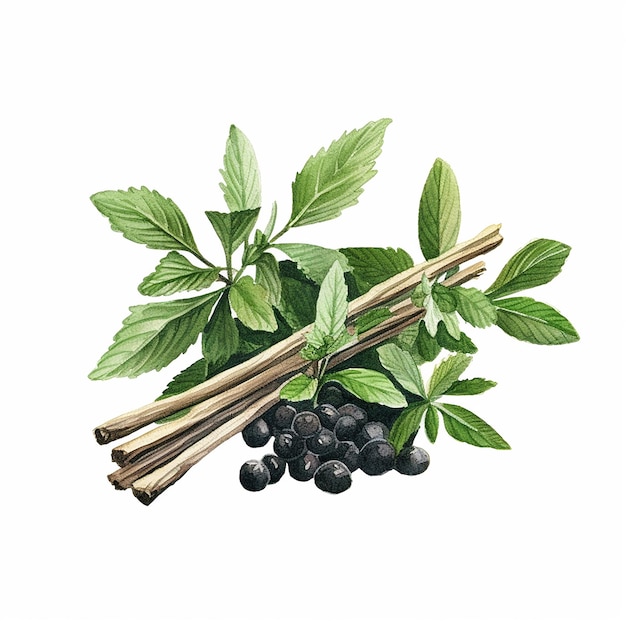The image is a highly detailed and brightly lit colored drawing, set against a solid white background, featuring green plants, dark berries, and several wooden sticks. The green plants have oval, pointy leaves with jagged edges that grow from green stems, adding a lifelike quality to the animated scene. In the center of the image sits a small mound of dark round berries that are a mix of black and dark purple—possibly blackberries or currants. Resting diagonally across the plants and above the berries are four thin, straight wooden sticks. These long sticks are light brown in color and angle up to the right. The clear, sharp details of the image emphasize its animated yet realistic style, free from any text or numerical elements.